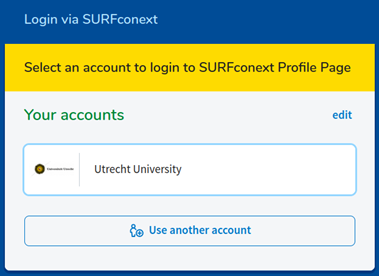The image is a screenshot of a login window from a specific website. At the top, there is a dark blue banner with the text "Login via SURF Connects" in white letters, with "SURF" and the "L" in "Login" capitalized. Below this, a yellow banner spans the entire width of the image, featuring black text that reads, "Select an account to login to SURF Connects profile page." The section beneath this displays a white background with the heading "Your Accounts" in light green on the left and an "Edit" option in blue on the right.

There are two rectangular sections below this. The first rectangle has a light blue border and a white interior with dotted lines on the left side, containing the text "Utrecht University" in black. The second rectangle, featuring the text "Use another account" in blue centered on a white background, is outlined by a blue border.

The entire login window is framed by a blue border that is visible on the top, left, right, and bottom edges of the image.